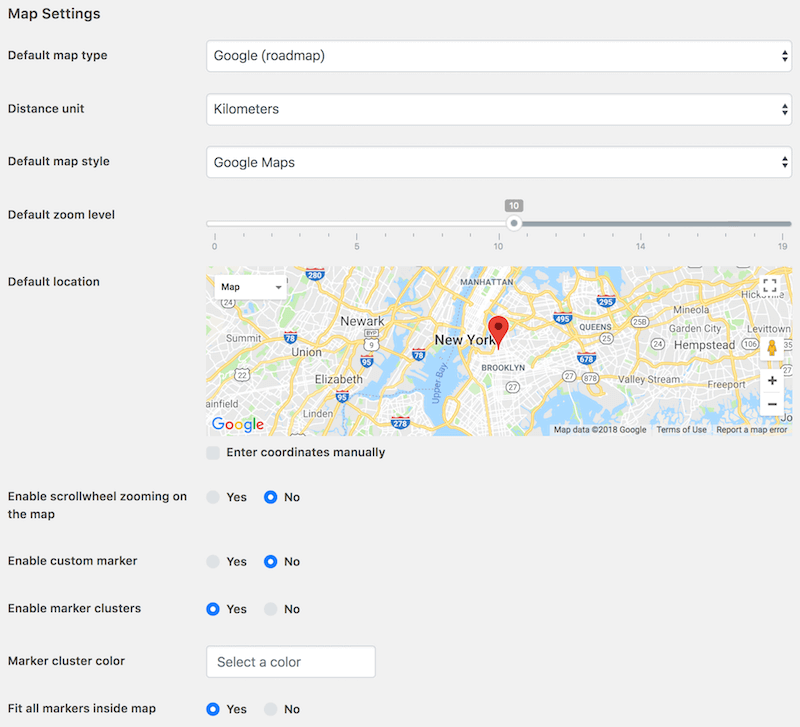The image depicts a detailed settings panel for configuring a map. On the left side of the panel, there are several options listed in sequence: "Map Settings," "Default Map Type," "Distance Unit," "Default Map Style," "Default Zoom Level," and "Default Location." After a few lines are skipped, additional options appear: "Enable Scroll Wheel Zooming on the Map," "Enable Custom Marker," "Enable Marker Clusters," "Marker Cluster Color," and "Fit All Markers Inside Map."

On the right side of the panel, the current settings are displayed: "Google Roadmap" for Default Map Type, "Kilometers" for Distance Unit, and "Google Maps" for Default Map Style. The accompanying visual shows a map of New York, which also includes parts of New Jersey and Long Island. There's a red location pin specifically placed in Brooklyn.

Further detailed settings under "Enter Coordinates Manually" are shown, with the following configurations: "Enable Scroll Wheel Zooming on the Map: No," "Enable Custom Marker: No," "Enable Marker Clusters: Yes," "Marker Cluster Color: Select a Color," and "Fit All Markers Inside Map: Yes." The settings panel meticulously outlines the customizable features available for tailoring the map's display and functionality.